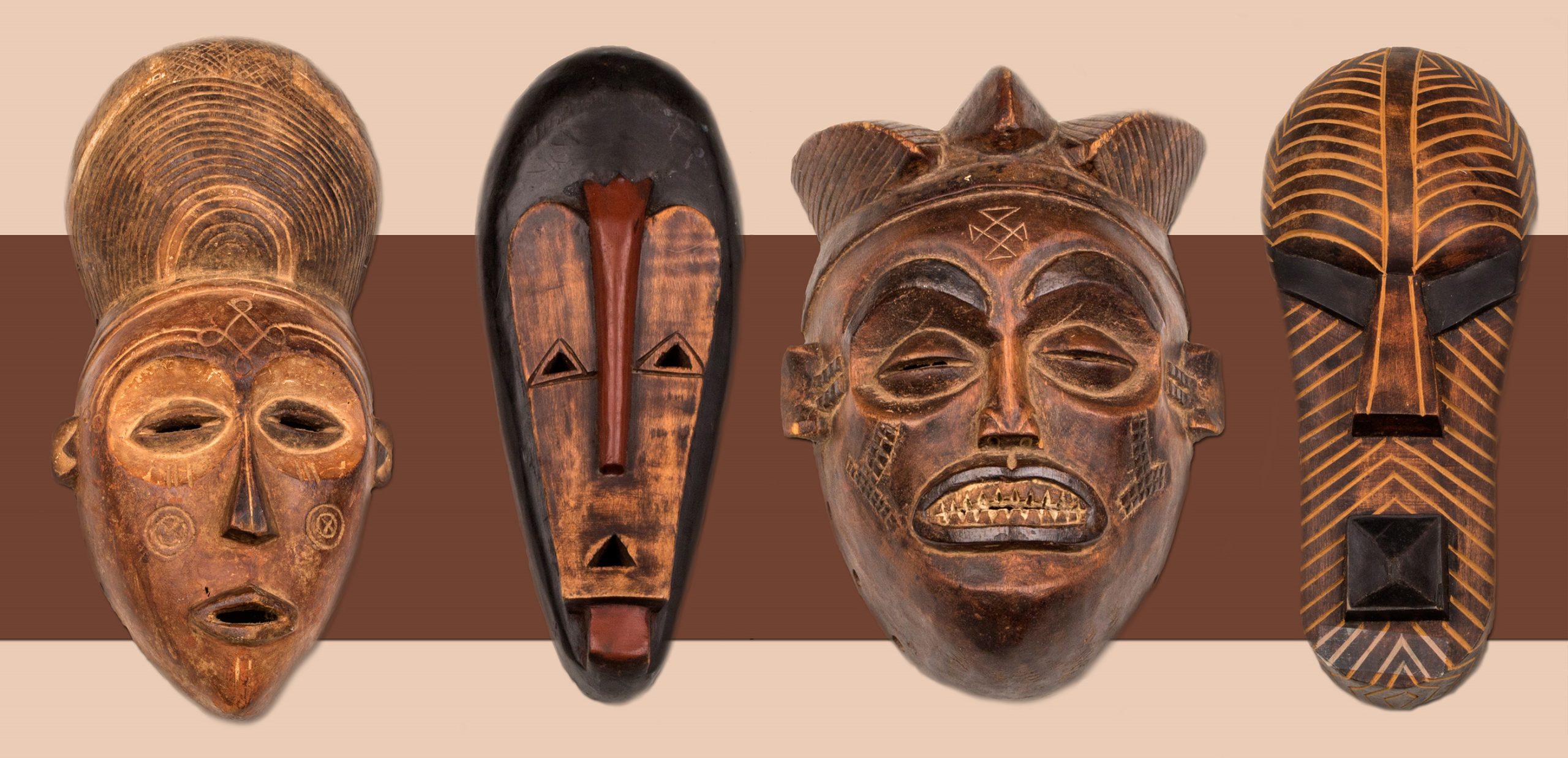This photograph showcases four distinct and traditional wooden masks displayed against a backdrop featuring a light tan or beige hue with a prominent brown horizontal stripe. The masks, varying in shape, color, and intricate details, exude an ancient, tribal essence.

On the far left, the first mask presents an almond-shaped head adorned with a rounded headdress. It features delicate marking circles on the cheeks and appears to be in a speaking position, adding to its lifelike quality.

The second mask, striking in its elongated teardrop-shape, is primarily black with a contrasting lighter brown face section. It is characterized by minimalist, geometric features—a triangle-shaped set of eyes and mouth, and a prominent dark brown nose.

Next, the third mask deviates from the elongated forms of its counterparts, exhibiting a more circular, coconut-like shape with a fuller, lifelike face. This dark brown mask showcases a three-sectioned spiky headdress, intricate facial markings, slit-like eyes, and a decayed appearance to its teeth, enhancing its uniquely foreboding aesthetic.

Lastly, the fourth mask boasts a long, narrow form with a striped pattern. The design includes brown with lighter brown lines radiating outward, coupled with simple black rectangular eyes and a black square mouth, giving it a stern and austere expression.

All four masks rest atop the brown stripe, creating a harmonious interplay of colors and textures against the muted backdrop while highlighting the diversity in their artistic and cultural representations.